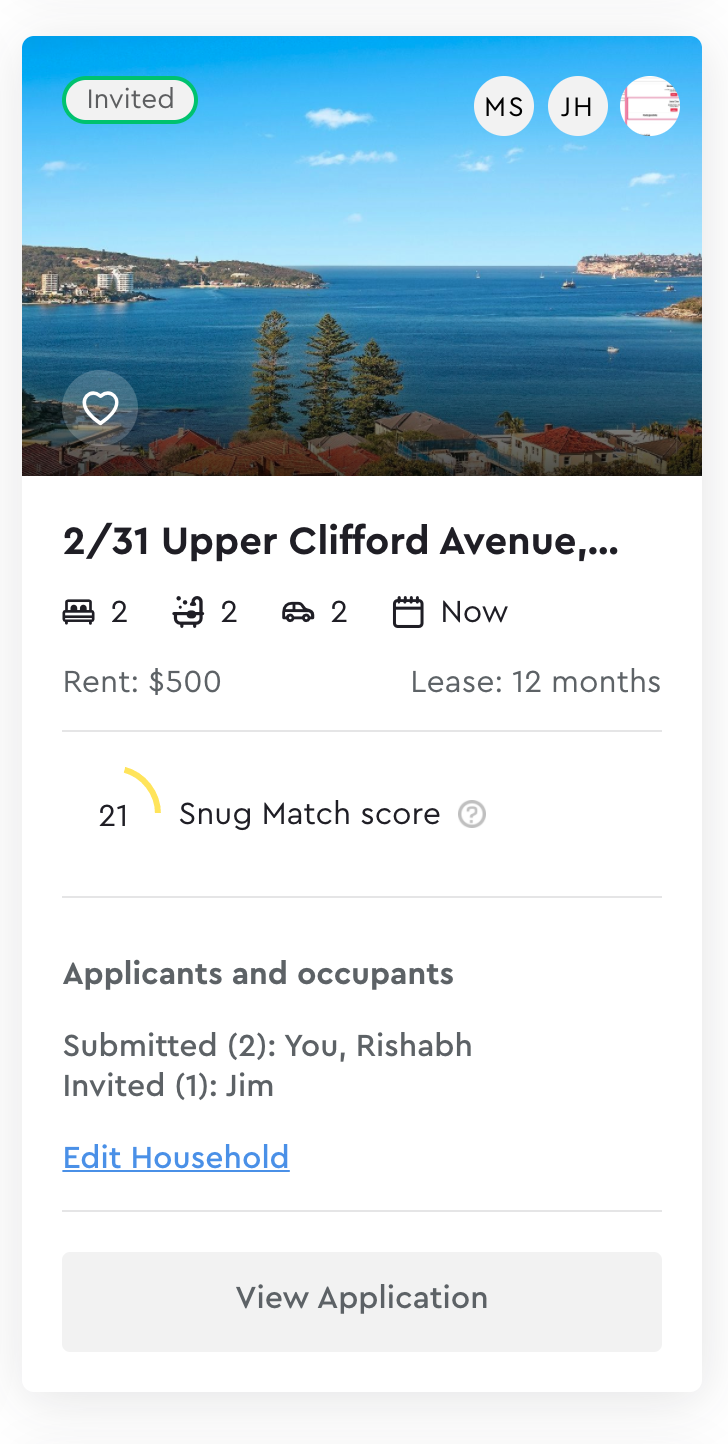**Detailed Caption:**

This image captures a detailed screenshot of a mobile app interface for an apartment rental listing, displayed on a cell phone. The orientation of the image is portrait, and it is set against a subtle white background with a faint gray outline around the edges, difficult to see but present. 

At the top of the screen, there is a landscape-oriented rectangular box showcasing a scenic view of a beautiful area with water, a clear blue sky, and land flanked by trees both to the left and right. This picturesque view is likely the immediate surroundings of the property.

In the upper left corner, a white chat bubble with a green circle containing the text "Invite" is visible, followed by several user icons: one labeled "MS," another labeled "JH," and a third icon featuring an unclear image.

Below the scenic image, the details of the property are listed:
- Address: **2-31 Upper Clifford Avenue**
- Key property features include: **2 beds, 2 baths, 2 car spaces**
- Availability: Marked with a calendar icon that says "Now"
- Pricing: **Rent $500, Lease 12 months**

A yellow meter below these details indicates a "Snug Match Score" of 21%, with the meter visually showing a 21% fill.

Further down, the section labeled "Applicants and Occupants" specifies:
- **Submitted**: "Two" names listed (You, Resheba)
- **Invited**: "One" name listed (Jim)

At the bottom of this section, there are options to "Edit Household" and "View Application."